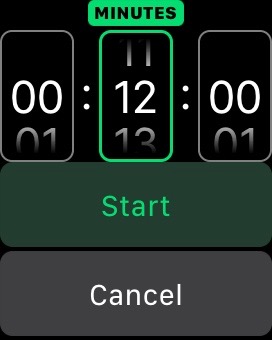This is a detailed screenshot of a timer app displayed on a smartphone. The app interface features a black background with white numerical text indicating the set time. The time displayed is precisely 00 hours, 12 minutes, and 00 seconds. At the top of the screen, there is a green banner with black text reading "Minutes." Below the numerical display, a bright green "Start" button signifies that the timer is currently running. Adjacent to the "Start" button is a gray "Cancel" button to stop the timer if needed. The sleek design and contrasting color scheme make the app user-friendly and visually appealing.